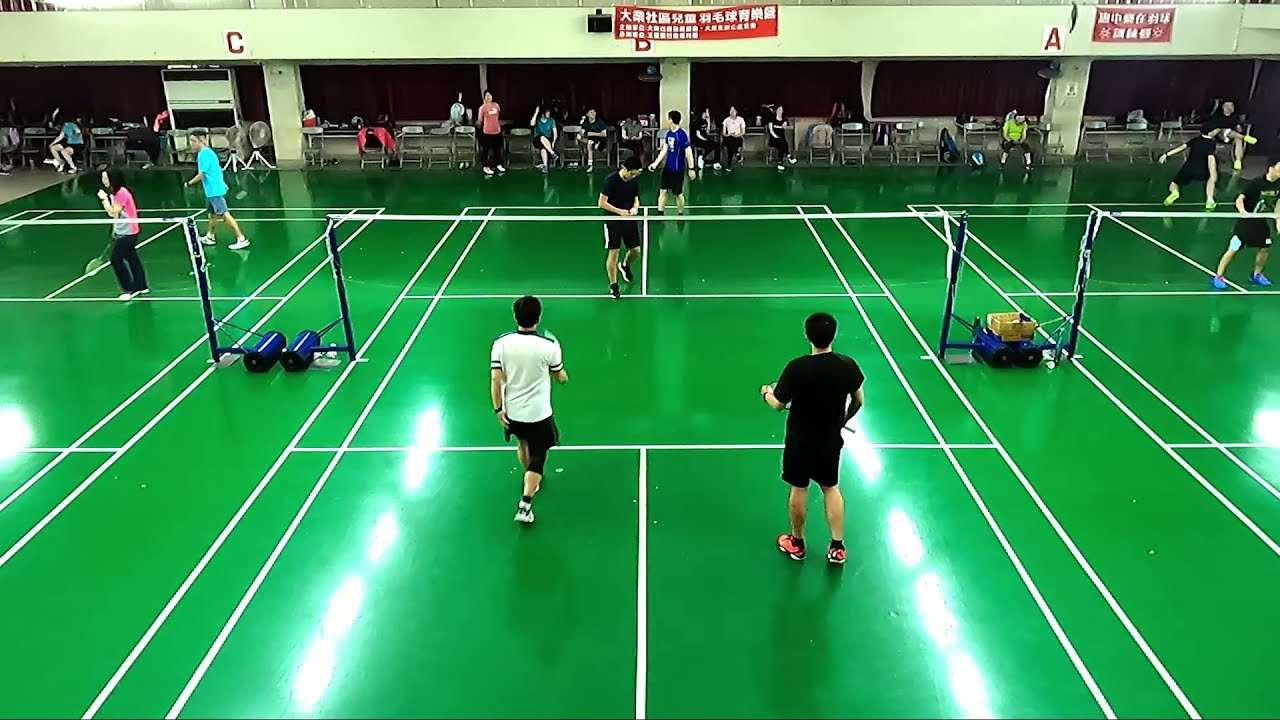The image depicts an indoor sports facility featuring three fully marked green courts, likely for badminton, given the white lines and the presence of nets held up by blue posts. Each court appears to be hosting a game, with doubles teams actively playing. The central court is entirely visible, while the two flanking courts are partially out of frame, showing only the players furthest from the net. The background reveals a black and yellow wall adorned with signage in Chinese, which hints at the possible location or cultural context of the facility. Additional spectators or participants are seated on folding chairs along the sidelines, and various tables are present in the distance. The overall scene captures a moment of multiple concurrent matches, suggesting a lively, competitive atmosphere.